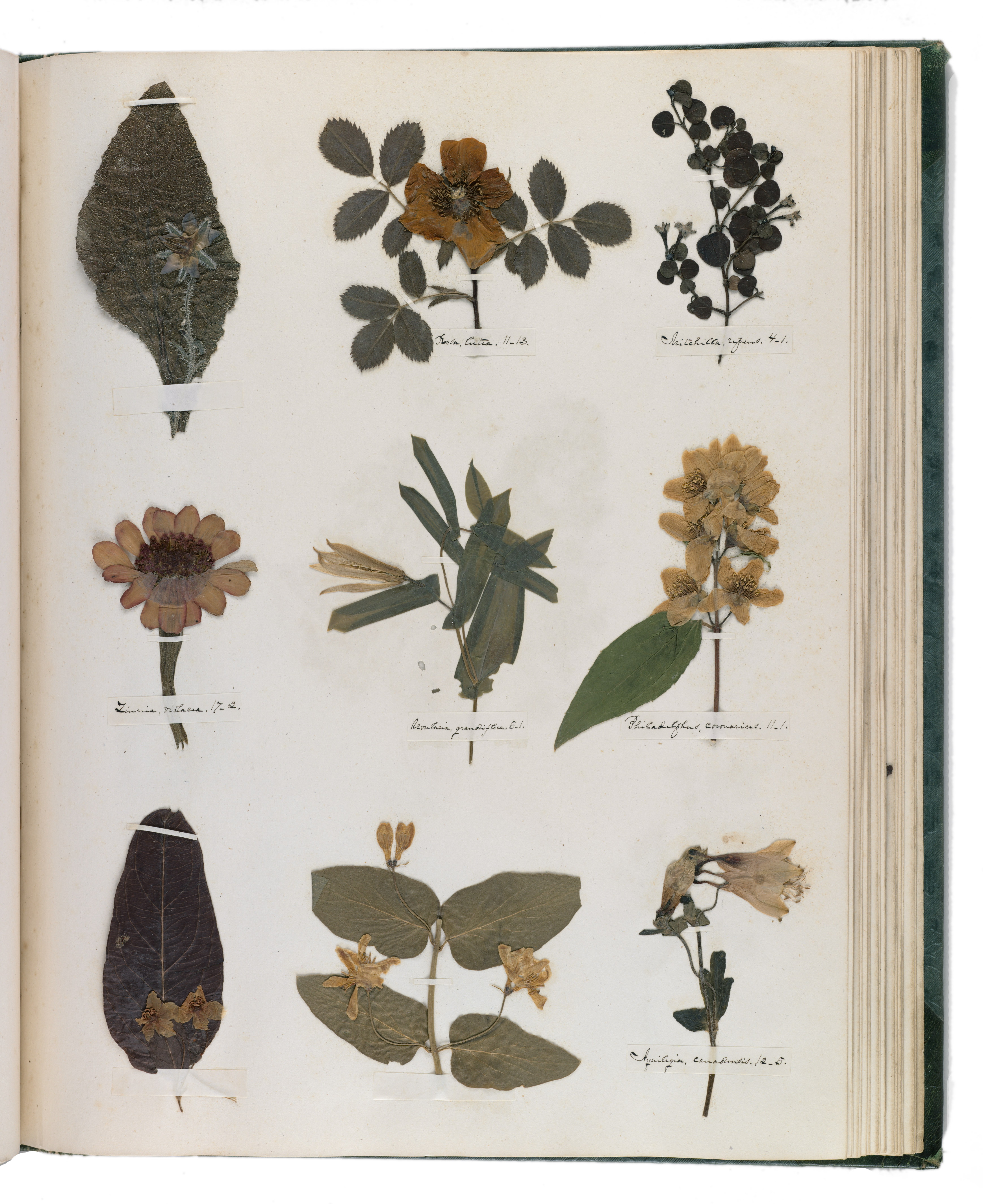This is a photograph of a book opened to a right-hand page displaying nine pressed botanical specimens, meticulously arranged in three columns. The left side of the book is mostly cut off, with only the center binding visible. The pages, made of creamy-colored, thin paper, have an aged appearance. Each specimen, consisting of leaves and flowering plants, is affixed to the page with labels beneath them—although the text on most labels is unreadable. One label reads "Julian Carrita, 11-13," and another specimen has a piece of white tape covering its title. The flowers, having lost most of their original color, exhibit varied hues of dark green and yellow-brown, indicating they have been preserved for a significant period. The varieties include different shapes and sizes, with one resembling an arrow and another showing a stem branching out with jagged-edged leaves. The samples are part of a larger collection within the hardcover book, distinguished by its dark green cover, visible along with several other pages in the background.